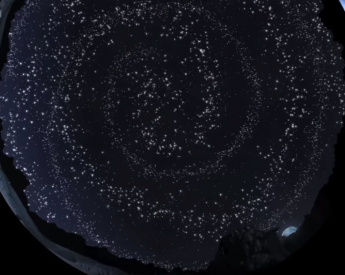The image depicts a stylized night sky rendered in a dark, nearly black, and deep indigo palette with hints of dark blue and purple. Dominating the center is a swirling pattern of countless bright white stars, evoking the appearance of a spiral galaxy or the Milky Way. This spiral, comprised of concentric circles, creates an illusion of depth and motion, with some stars appearing as more prominent flecks of light. In the bottom left corner, a small lake and patch of land are subtly visible, adding to the scene's atmospheric depth. The bottom right corner features a silhouette of a mountain, partially overshadowed by the night, and a half-visible moon tinged with light blue and dark blue spots. The image's quality is relatively low, contributing to a more abstract and artistic impression rather than a detailed photograph, yet it encapsulates a sense of cosmic wonder.